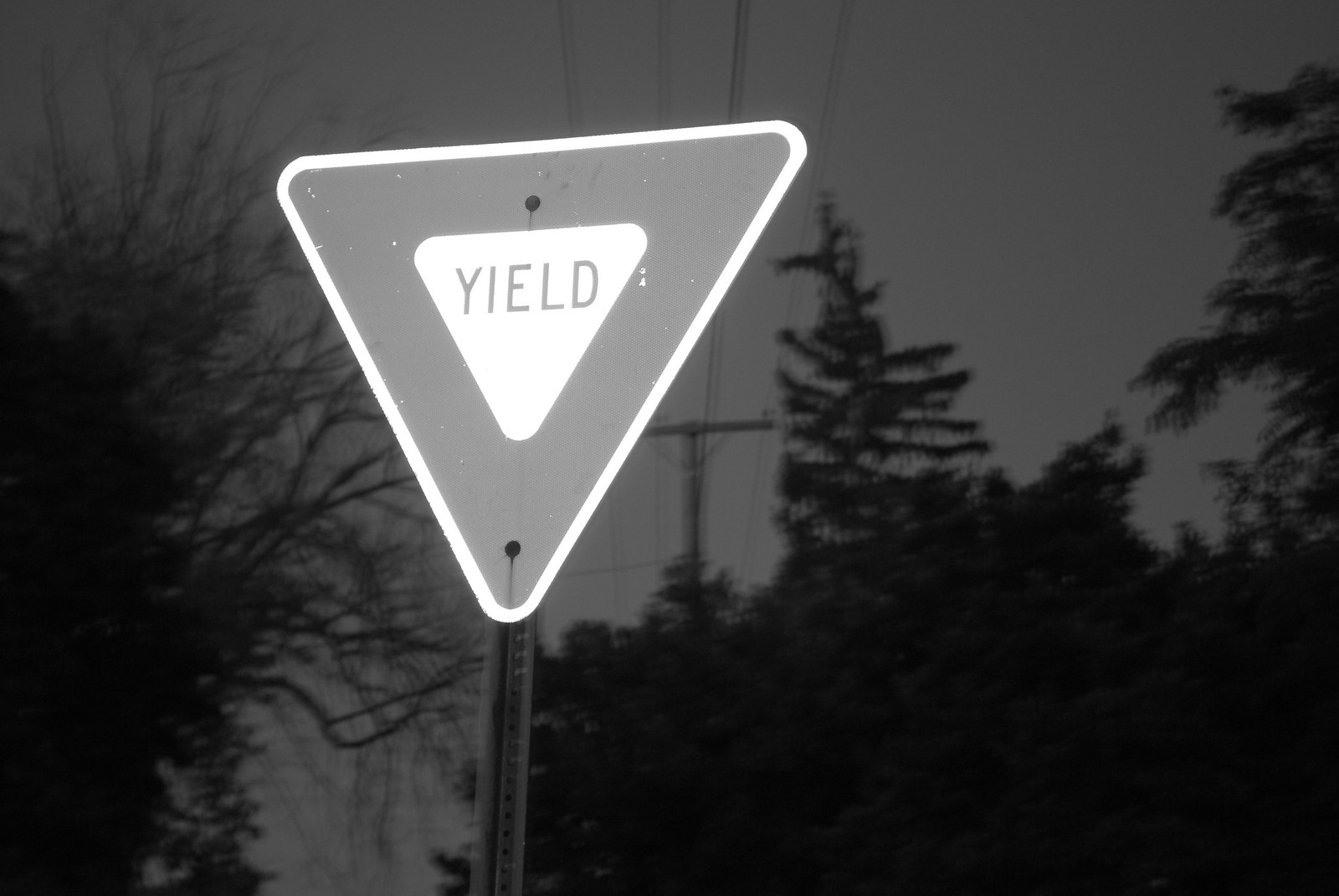In this striking black-and-white photograph, a prominently reflective yield sign commands attention against a dark, indistinct background. The yield sign, affixed to a metal pole with two large rivets, has a slightly weathered appearance with minor dents and scratches particularly around its edges. It is an upside-down triangle with a glowing white rim, a darker inner field, and a white center displaying the word "YIELD." The sign's reflective surface almost illuminates, contrasting sharply with the dim surroundings, suggesting it is nighttime. Behind the sign, dark and somewhat out-of-focus trees can be seen on both sides, including a spindly tree to the left and more typical pine trees to the right. Furthermore, utility poles and electrical wires are visible near the trees, adding to the image's stark and utilitarian scene. The photograph masterfully highlights the yield sign, emphasizing its brightness and functionality in low-light conditions.